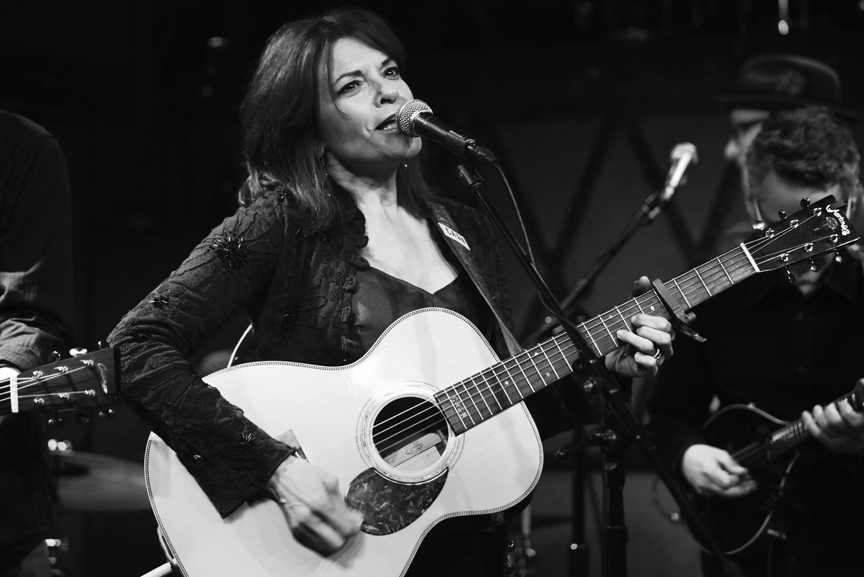In a timeless black and white photograph taken during a concert, a captivating female singer takes center stage. She stands with short dark hair, wearing a long-sleeved blouse paired with a dark shirt underneath, her attire textured like flowers. The singer's head is tilted slightly back, her mouth open as she pours her soul into a song. Her left hand grips the wooden neck of an acoustic guitar, holding it diagonally with the neck positioned to the right side of the image. Her right hand is caught in motion, strumming the strings downward.

The microphone stands prominently in front of her, angled slightly downward. Behind her on the right-hand side, there is a person with short curly hair playing a ukulele; their face mostly hidden by the lead singer's guitar. Another musician is partially visible, wearing a short boulder cap and talking into a standing microphone. There’s also the hint of another person cropped out on the left-hand side. The backdrop, slightly out of focus, frames the scene, capturing the essence of live music and the camaraderie of the performers.